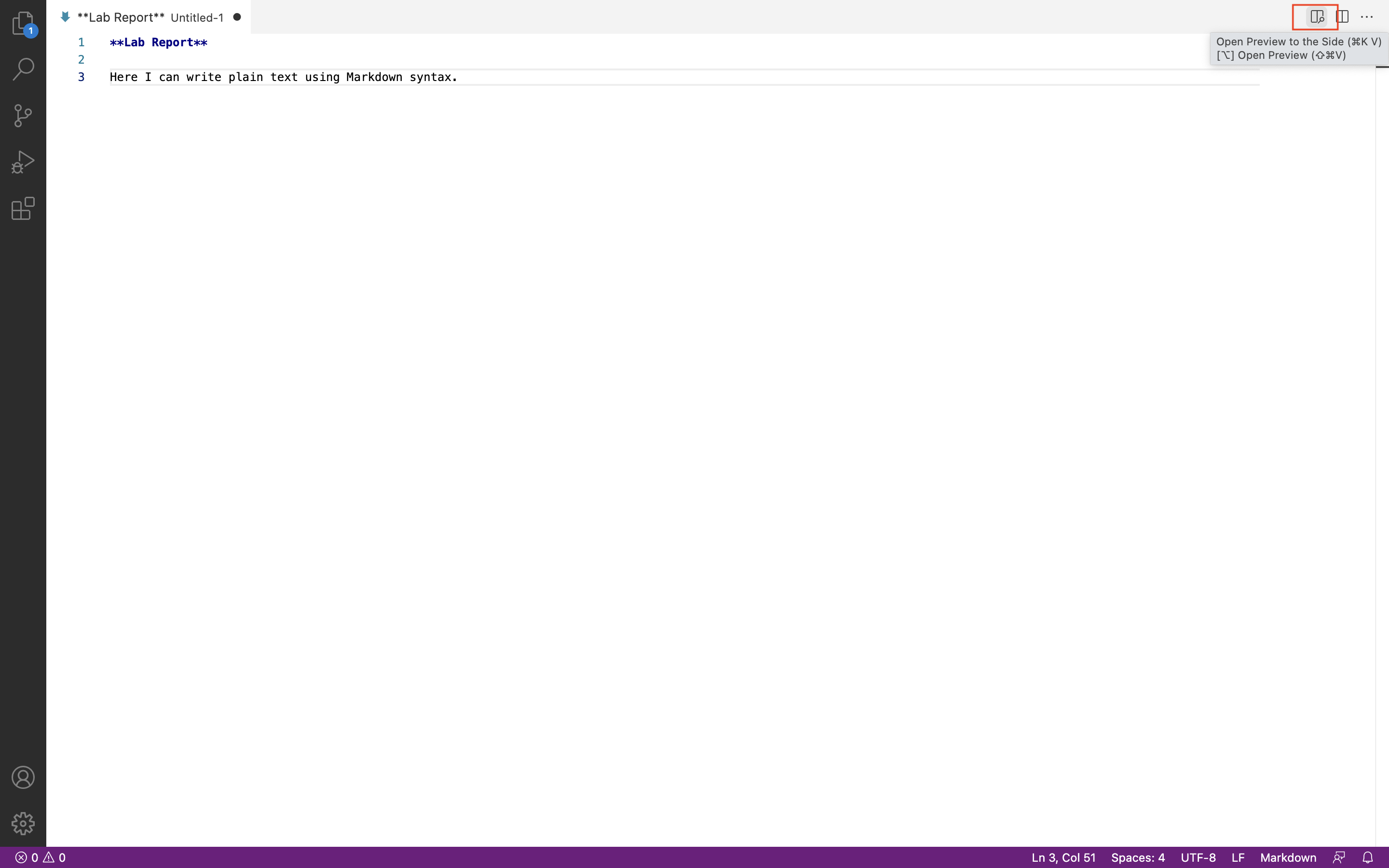This image showcases a computer screen displaying a mostly blank, white document in a program. In the top left corner, there are several option icons: a magnifying glass for search, two overlapping papers indicating duplication or copying, and a triangular play button pointing to the right, likely for executing a command or previewing the document. In the bottom left corner, a settings icon resembling a gear is visible, alongside a profile button depicted as a forward-facing person.

On the top right corner, there is a small red square highlighting one of the options. At the very bottom of the screen, a thin, purple taskbar stretches across, filled with white text descriptions that are very small and located towards the bottom right corner.

In the top left part of the screen, there is an open tab titled "Lab Report, Untitled #1". Directly below this tab, the text reads "Lab Report" with the instruction: "Here I can write plain text using markdown syntax".